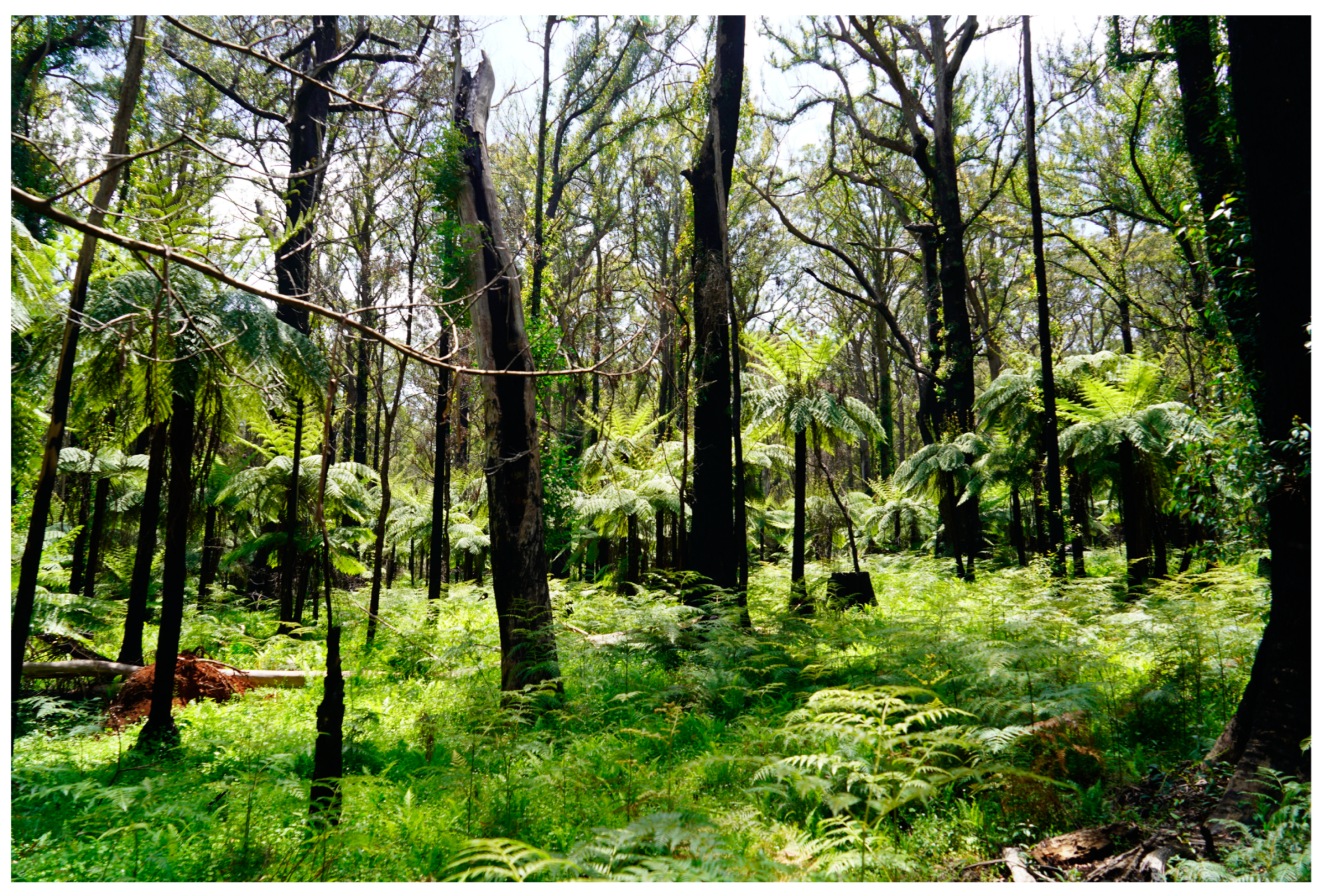The photograph captures a lush, green, and slightly overgrown woodland environment, evocative of a rainforest. Despite the image's blurriness, it's clear that there are numerous tall and skinny palm trees, with their tops displaying empty branches. The forest floor is densely covered in various ferns, grasses, and other plants, showcasing a vibrant and rich green palette that hints at the spring season. Additionally, some trees appear to be cut or fallen, particularly noticeable in the bottom left-hand corner of the frame, where there are scattered branches. The overall scene is sunlit, with shadows cast on the greenery and a bluish-white sky visible in the distance. This natural setting, possibly resembling the Midwest or even an Amazonian jungle, gives off a serene yet slightly abandoned feel with no visible animal life, just the diverse and thriving plant life.